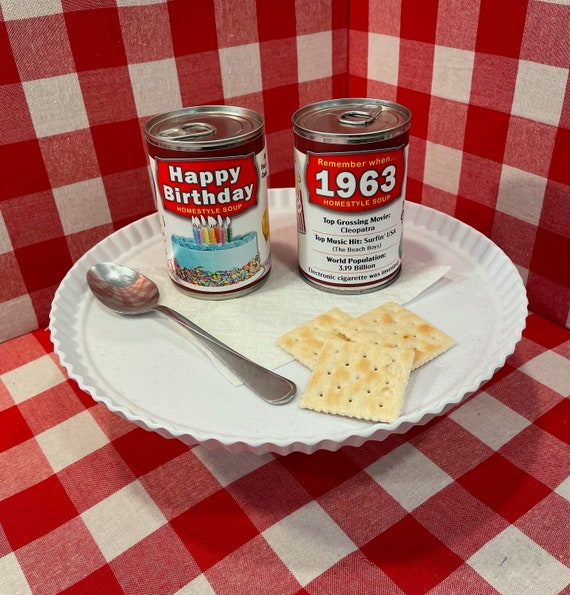This indoor photograph captures a white china plate set in a corner, enveloped by a red and white plaid cloth covering the bottom, surface, and both walls of the corner. Resting on the plate are two aluminum soup cans, accompanied by a stainless steel spoon on the left and three beige, square-shaped saltine crackers on the right. A white napkin lies beneath the cans. The cans are distinctly labeled: the one on the left reads "Happy Birthday Home Style Soup" with a graphic of a blue birthday cake adorned with multicolored sprinkles and lit candles. The can on the right features a nostalgic label that reads, "Remember when 1963, Home Style Soup," alongside historical trivia including "Top Grossing Movie: Cleopatra," "Top Music Hit: Surfing USA, The Beach Boys," "World Population: 3.9 Billion," and "Electronic Cigarette was invented."